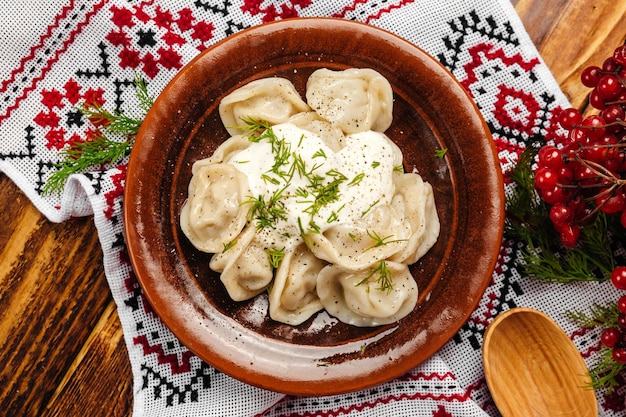In this image, we observe a rustic wood table adorned with an intricate, mostly white embroidered cloth featuring symmetrical red floral details with black centers and black V-shaped stitching. Centered on this cloth is a deep, rustic brown bowl containing numerous tortellinis of a very light brown, almost whitish hue. The pasta is generously topped with what appears to be Alfredo sauce and garnished with green herbs. To the right of the bowl, additional garnishes, resembling bunches of mistletoe with red berry-like accents and green leaves, are scattered on the table. At the bottom of the frame, a wooden spoon with a light green and brown handle peeks into view.